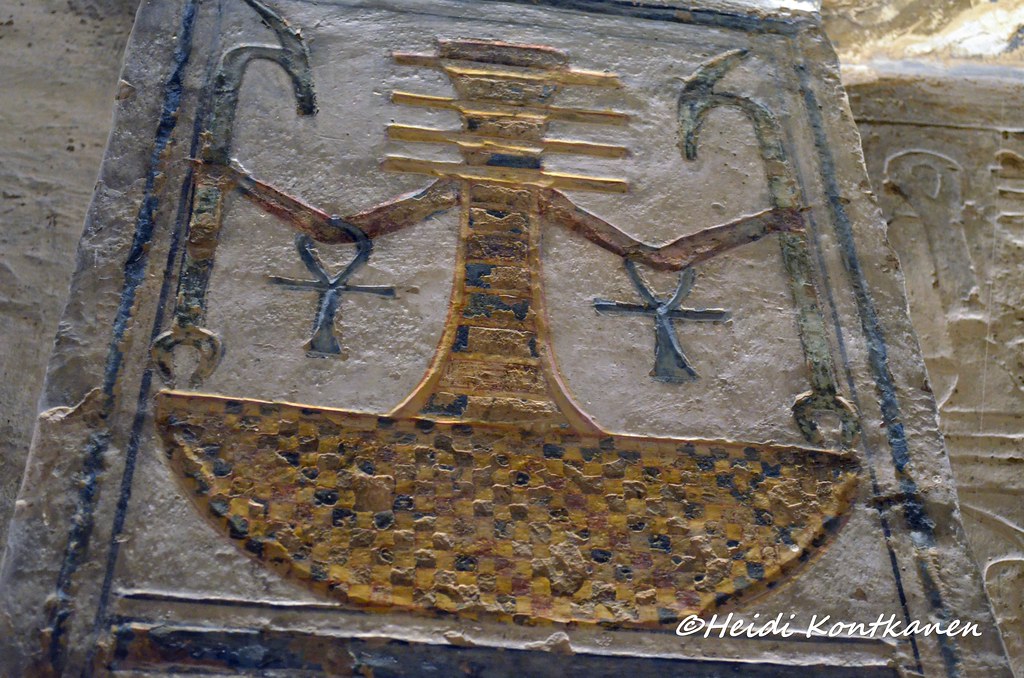The image is a horizontally aligned, rectangular close-up of an intricately designed stone artwork, likely on a monument or a building. The central square area of the stone features a character that appears to be inspired by Egyptian hieroglyphics. The figure has arms extended outwards, with blue and gold checkered elements hanging from the elbows. The figure’s lower body transitions into a basket-like pattern, intricately woven in gold with alternating brown and navy squares. Horizontal gold slashes adorn where the head should be, giving it an abstract aesthetic. A blue border frames the central area. On the right side of the stone wall, there are additional carvings that seem to depict a goose's neck and head. The left side shows a textured brown-tan mix of stone. Near the bottom right corner of the artwork, there's a copyright symbol along with the artist's name, Heidi Cont Cannon. This combination gives the entire piece a vivid mix of ancient and modern artistic elements.